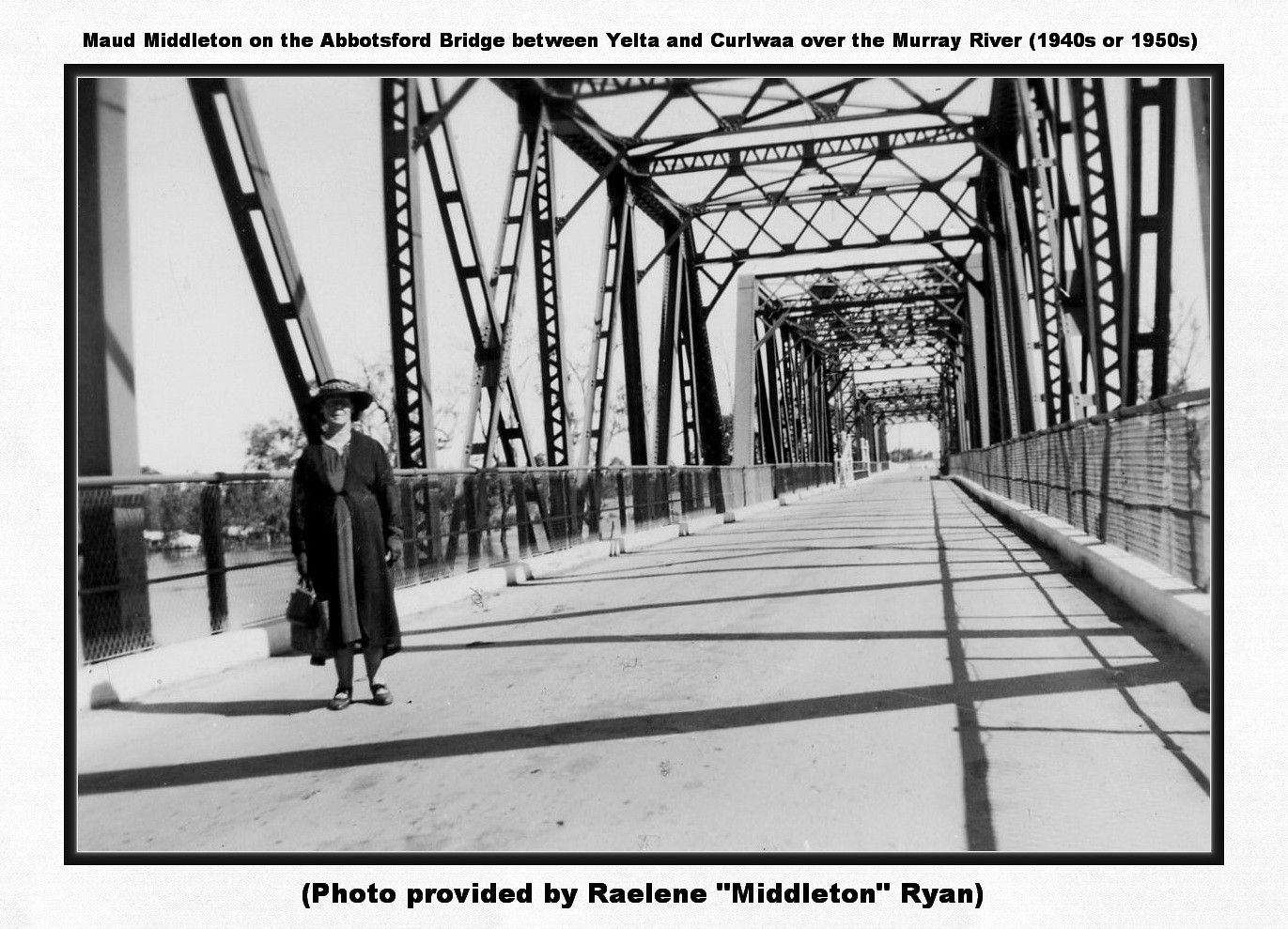This detailed black-and-white photograph captures Maude Middleton standing on the Abbotsford Bridge between Yelta and Curlewa over the Murray River, likely taken in the 1940s or 1950s. Positioned on the left side of the image, Maude is attired in a dress that falls below her knees, complemented by a long overcoat. She wears dark shoes and a prominent dark hat adorned with a lighter-colored band. She holds bags in her right hand, with both hands resting by her sides. The bridge features two shoulder-height fences on each side and is framed by extensive metal framework that occupies the top half of the image. The photograph has a black border followed by a light blue one. At the top of the border, bold black text reads: "Maude Middleton on the Abbotsford Bridge between Yelta and Curlewa over the Murray River, 1940s or 1950s." A bottom text states: "Photo provided by Raylene Middleton Ryan." The bridge stretches into the distance, accentuating its vast, structural elements against the stark monochrome backdrop.